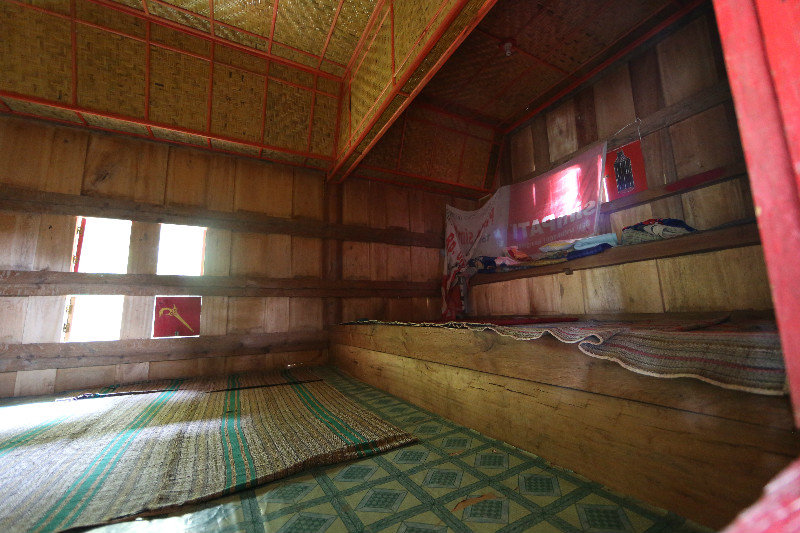The image depicts an interior of a room that resembles a traditional building possibly used for religious or educational purposes. The room is primarily empty of furniture, but the floor stands out with its green tiles featuring various shades of green arranged in a diamond pattern, although some tiles exhibit wear and tear, suggesting it might be linoleum. 

A striped carpet in shades of blue, red, brown, and green lies folded over in one part, allowing a glimpse underneath. The walls are constructed of wood planks, and there are multiple window openings. One such opening is covered by a red cloth with an embroidered golden design, which appears to be an umbrella or another intricate pattern, though it's hard to discern. 

On the right-hand side of the room, there's a stage-like platform with a red and green striped carpet and a reddish-pink curtain hanging nearby. Items such as towels, folded on a wooden bench, and possibly backpacks or packs placed on a ledge, are scattered around the room. The ceiling features a woven or thatched look, possibly made from bamboo or wicker, with a grid of red or orange bars crisscrossing it.

In the background, several flags and posters, predominantly red and white, are hung alongside some wooden steps outfitted with pillows, suggesting a seated area. Overall, the room's design, with its wooden elements, intricate ceiling, and varied floor and wall decorations, evokes a warm and traditional ambiance, reminiscent of a sauna or a clubhouse.